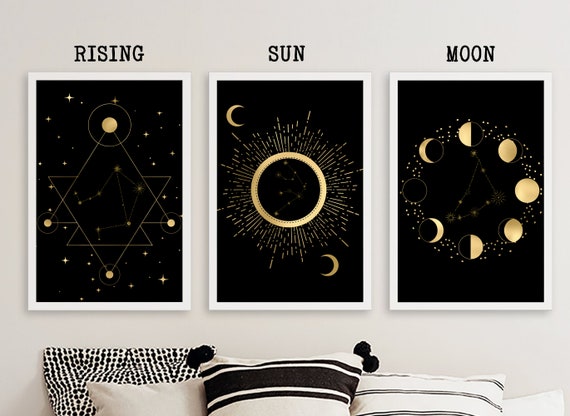This photograph, likely from an online catalog, showcases a stylish home decor arrangement featuring both modern art and chic throw pillows. The bottom of the image displays four black-and-white patterned throw pillows. From left to right: the first pillow is square and white with black polka dots; the second, smaller pillow is pure white; the third pillow, also white, boasts broad black stripes flanked by narrower stripes and is adorned with black pom-pom fringes at the corners; the fourth pillow is white with double narrow black stripes running across it. 

Above the pillows, set against a light gray wall, are three framed prints, each with a solid black background and white frame, arranged in a vertically oriented rectangular (portrait) layout. Evenly spaced black capital letters above the frames label each print: "Rising," "Sun," and "Moon" from left to right. The "Rising" print features what appears to be a constellation with intersecting lines and geometric patterns in gold. The "Sun" print depicts a starburst design with a central black circle surrounded by gold lines and crescents. The "Moon" print illustrates the moon's phases arranged in a circular pattern, all rendered in gold. The cohesive black-and-white color scheme with touches of gold unifies the decor, creating an elegant and harmonious visual appeal.